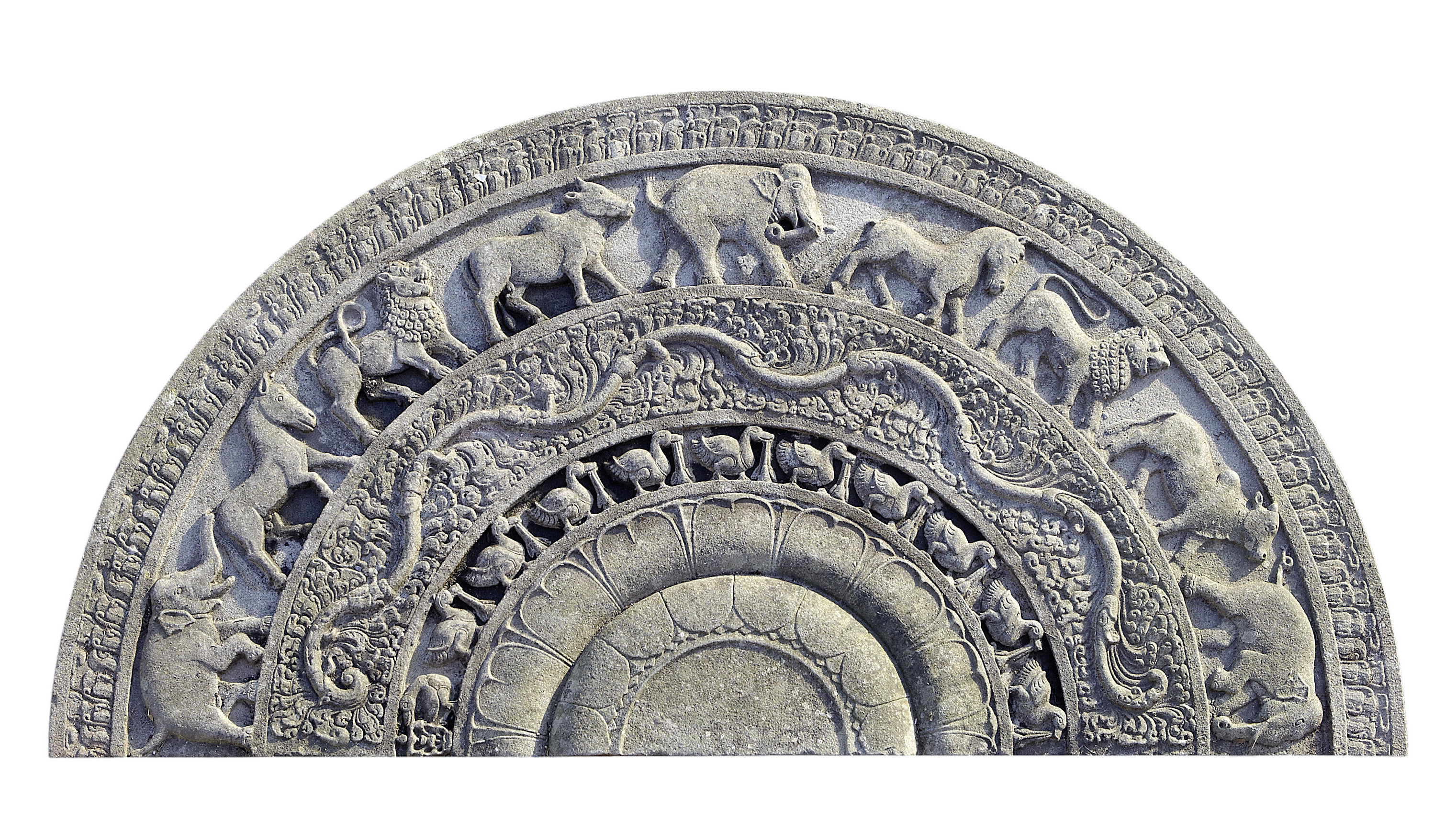This photograph captures the top half of an intricately carved round stone, possibly from ancient times such as Greek or Roman eras. The stone, rendered in a light gray color with some sections appearing black, features detailed engravings of various animals in a circular arrangement. The animals include an elephant, a horse or donkey, a lion, and a cow, which repeat in sequence around the stone's perimeter. Beneath the animals is a snake-like or vine-like design, followed by a ring of duck or dove carvings. The stone appears to stand upright with the flat cut edge at the bottom, and it is set against a solid white background, highlighting its detailed craftsmanship. The image suggests the stone could be part of an ancient tomb or mausoleum, showcasing its historical and artistic significance.